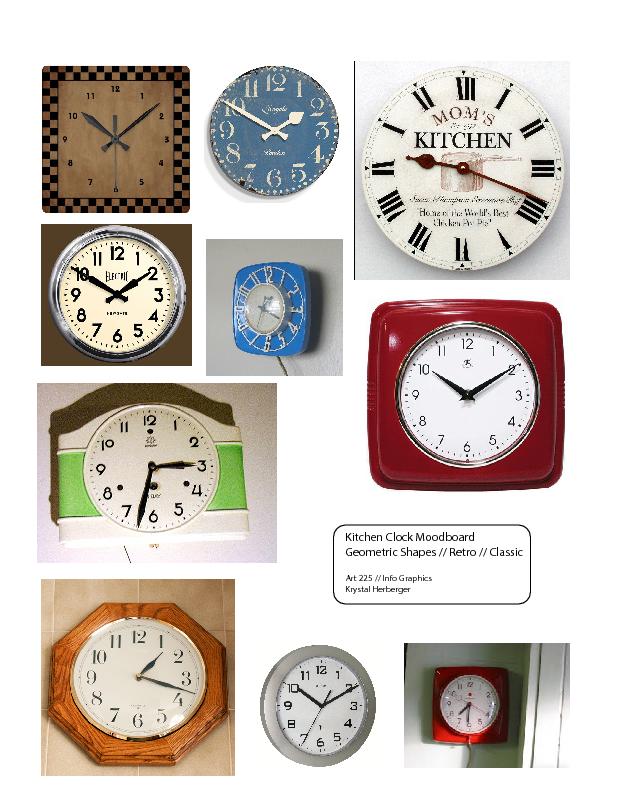The image captures a collage of ten diverse clocks arranged in a grid-like format. This mood board includes various geometric shapes and styles, both retro and classic. The clocks showcased encompass a range of designs, from a wooden square clock with a checkered border in the top left, to an octagonal wooden clock in the lower left corner. There's also a red square clock with a white face displaying black numbers and hands. Prominently featured is a circular silver clock, and another notable clock is a white one inscribed with "Mom's Kitchen" in red and black letters, although part of the text is unclear. An ornamental green and white clock is among the collection, alongside a regular round silver clock. Notably, one of the clocks uses Roman numerals. The image also includes a white bordered rectangle text box located at the bottom right, stating "kitchen clock mood board geometric shapes retro classic art 225 infographics" and some additional, partially obscured text. This assemblage appears thoughtfully curated to display a variety of kitchen clock styles and inspirations.